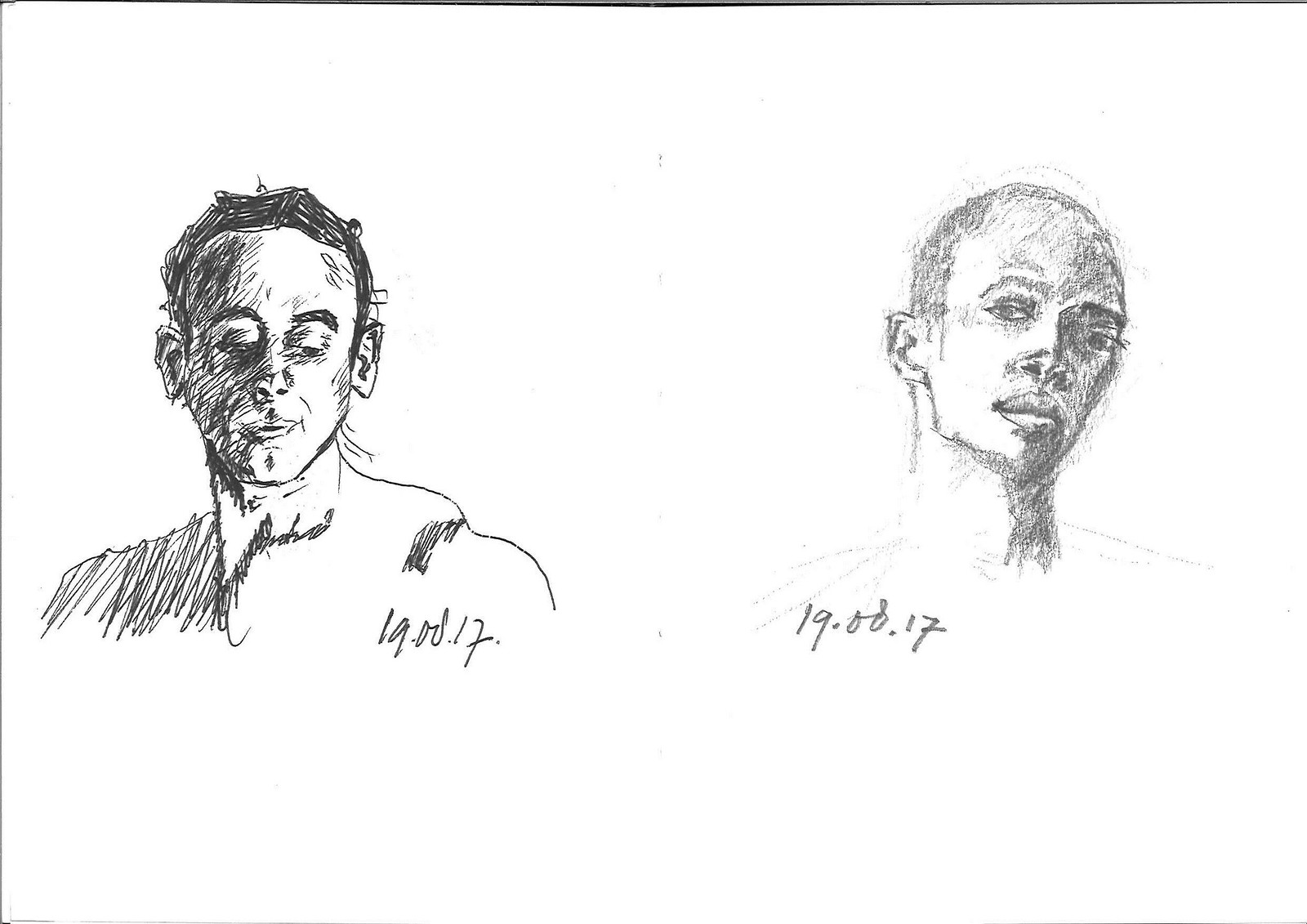The image features two detailed sketches side by side, each showcasing a bust of a man. 

**Left Sketch:**
The left sketch is created using black pen, depicting the bust of a Caucasian man. He has short, cropped hair and is looking downward to his left (our right), with his eyelids partially closed. His hair is heavily shaded in dark pen strokes. The right side of his face (our left) and parts of his neck also exhibit strong, dark pen lines, contributing to the overall shading and depth of the sketch. His attire is indistinct, but there are various levels of shading throughout the bust. Below his left shoulder (our right), the numbers "19.00.17" are written.

**Right Sketch:**
The right sketch is done with a lead pencil, illustrating the bust of an African man. He is looking directly ahead, with a slight tilt of his head to his left (our right). He features short, cropped hair and a goatee beard. The pencil strokes are much lighter compared to the pen sketch on the left, resulting in a softer, more subdued depiction. Similarly, the numbers "19.00.17" are written below his right shoulder (our left).

The contrast between the bold, dark pen lines on the left and the soft, delicate pencil strokes on the right highlights the distinct techniques and brings a unique character to each sketch.